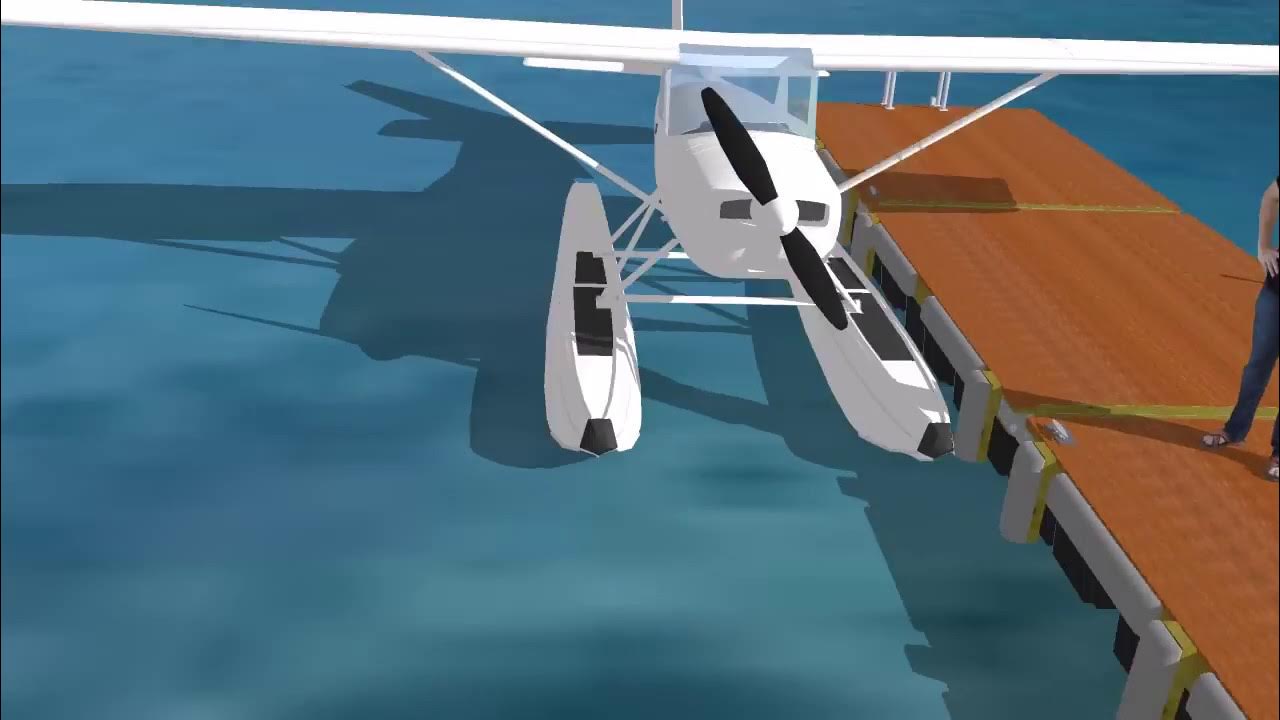This rectangular, digitally generated image, approximately six inches wide and three inches high, depicts a seaplane docked on blue water. The seaplane, which is white with a black propeller, is positioned towards the center-left side of the image, with its propeller facing the viewer. The dock extends diagonally from the lower right-hand corner, featuring light brown decking supported by gray pillars. A person, wearing blue jeans, is partially visible on the right edge of the image, with their right arm resting on their hip. The individual appears to have a Caucasian skin tone. Shadows cast by both the person and the plane add depth and realism to the scene, despite its overall animated and somewhat stylized appearance. The setting suggests a private seaplane loading zone, rendered with detailed attention to the water's varying shades of blue and the precise placement of elements within the frame.